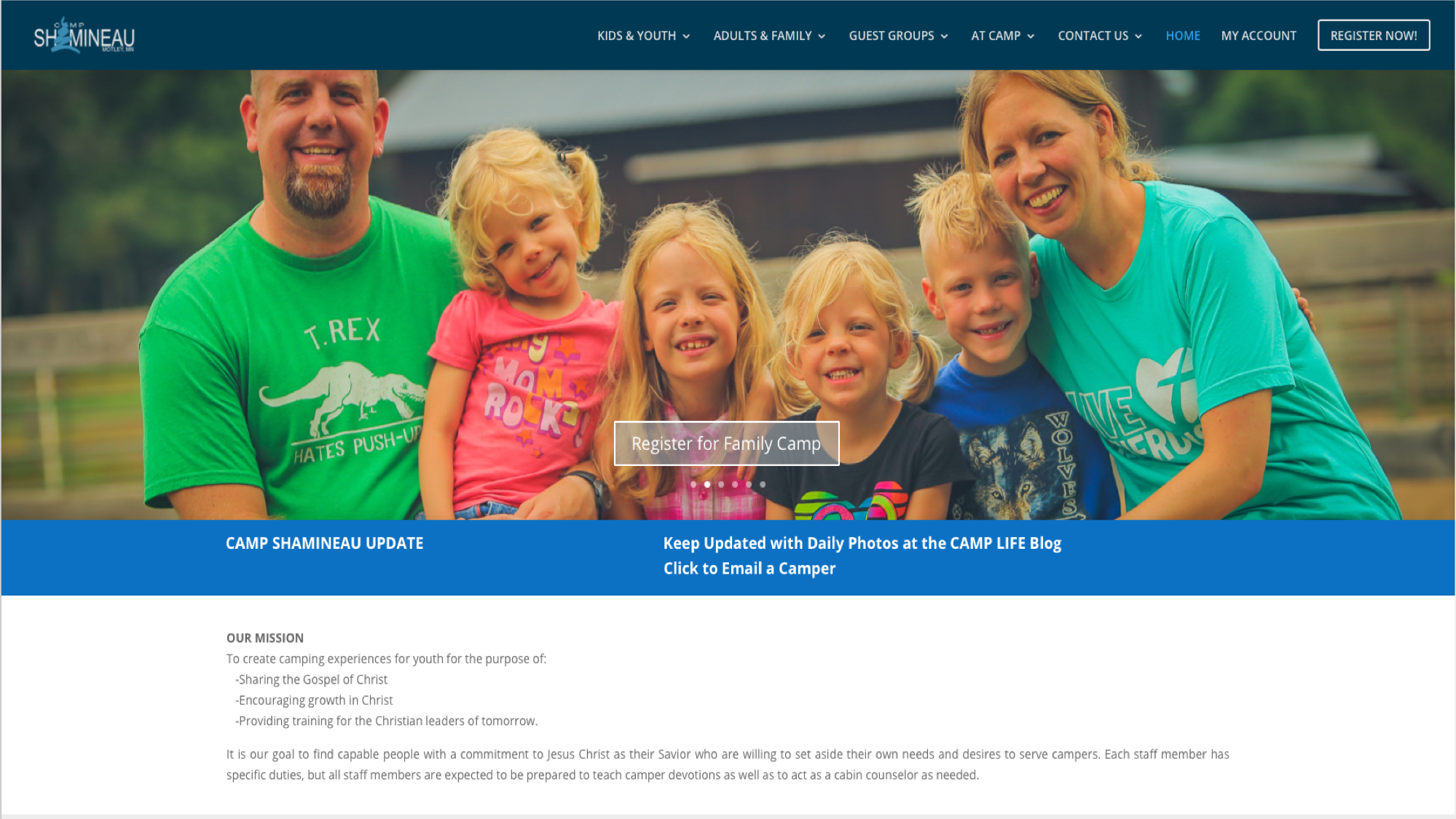The image showcases a website header against a dark navy blue background with the brand name "Chimeno" prominently displayed in the top left corner. Along the top right are several clickable drop-down menus labeled: Kids and Youth, Adults and Families, Guest Groups, At Camp, Contact Us, Home, and My Account. A "Register Now" button, matching the background color but bordered with a white rectangle and with the text in bold white capital letters, is prominently featured. 

Below the header, an outdoor photograph captures a serene scene with trees in the distance and a wooden fence marking the area. In the background, a structure is partially visible. Foregrounded are four individuals: a chubby man on the left with a goatee, wearing a green shirt featuring a dinosaur and the humorous text "T-Rex Hates Push-Ups"; next to him stands a young girl in a pink shirt with blonde hair; followed by another blonde-haired girl in a purple shirt; and lastly, a girl with blonde hair and a black shirt.